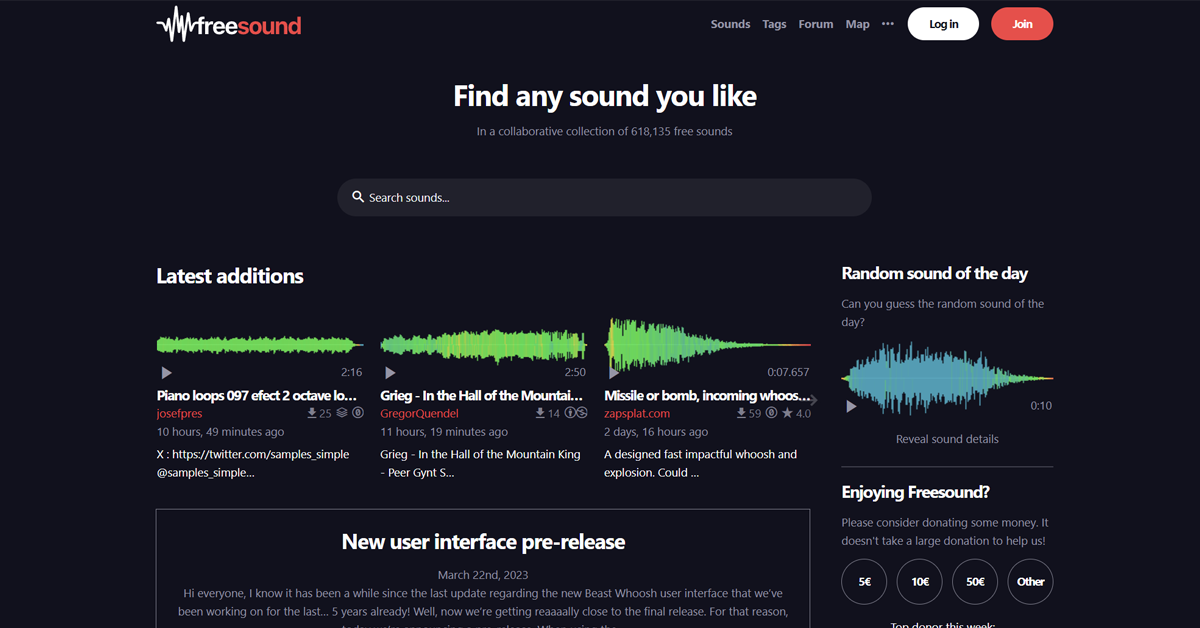This image captures a landscape-oriented screenshot of a web application set against a black background, approximately twice as wide as it is tall. At the top of the interface, there is a distinct icon followed by text with the first part in white and the second part in red. This icon and text form the name "Free Sound". 

To the right of this name, there are several navigation options displayed in white text: "Sound Tags," "Forum," and "Map". Close to these, there are two buttons – a white "Login" button and a red "Join" button written in white font.

Below the navigation bar, a prominent white header reads, "Find any sound you like," along with a subtext in white indicating, "in a collaborative collection of 618,135 free sounds." Beneath this is a gray search bar with white lettering. Following the search bar, there is a section titled "Latest Additions" in white text, showcasing clickable sound thumbnails. Each thumbnail features green sound wave imagery, along with headings and titles underneath in a mix of white and red text, also indicating the submission times.

At the bottom of the image, there is a thin white border framing a section that announces, "New User Interface Pre-Release," accompanied by additional explanatory text beneath it.